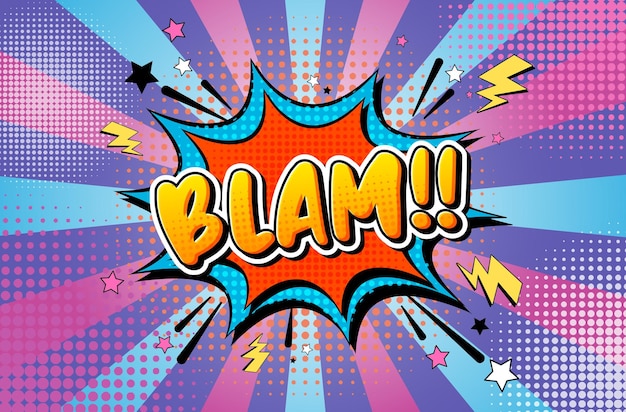This digital cartoon image features a dynamic, comic book-style design reminiscent of old Batman TV shows. At the center, the word "BLAM!!" is prominently displayed in vibrant yellow bubble letters with an orange outline, evoking a sense of explosive action. This central text is surrounded by a splat shape comprising a mix of blue and orange splotches, with orange dots scattered around the edges, enhancing the chaotic visual impact. Surrounding the "BLAM" are additional elements such as yellow lightning bolts and pink and white stars, which amplify the comic book aesthetic.

The background radiates out in a starburst pattern, with straight lines in vivid hues of pink, purple, and blue shooting diagonally from the center, creating a noisy and energetic atmosphere. The lines resemble the American flag's stripes but are arranged diagonally, converging towards the central "BLAM." This composition not only highlights the explosive main text but also contributes to the overall lively and eye-catching visual style of the image.